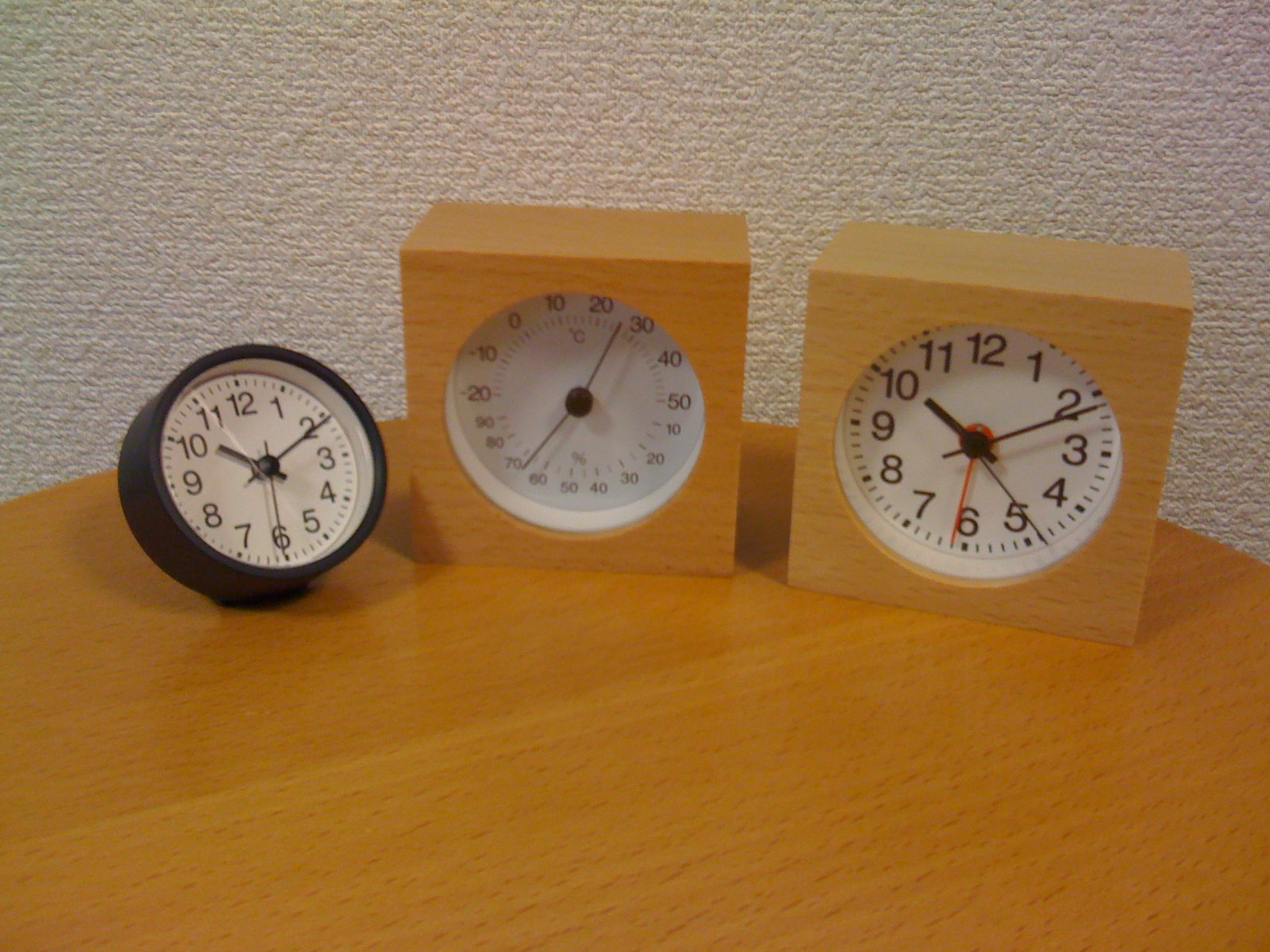This image features a trio of distinctive timepieces arranged on a tan or very light oak table, possibly resembling a pine finish. The backdrop appears to be a white, textured wall, reminiscent of a hotel room's interior.

1. **Round Black Alarm Clock**: To the right, there's a classic round black alarm clock with a white face. It boasts bold black hour and minute hands, along with a thinner black second hand. The hour hand points to 10, the minute hand to the 2, indicating a time of 2:10. Notably, this clock rests at a slight backward tilt rather than standing upright.

2. **Square Temperature Gauge**: Adjacent to it, there is a square temperature gauge made of a material that matches the table’s oak-like hue, darker than pine. This device is not a clock but a thermometer displaying temperature in both Celsius and Fahrenheit. It features two scales: one for Celsius, ranging from -20 to +50, and another for Fahrenheit, ranging from 10 to 90, with intermediate markings. The hands of the gauge point approximately between the 20 and 30 degrees Celsius mark and between the 60 and 70 degrees Fahrenheit mark.

3. **Pine Wood Travel Clock**: On the far left, a lighter wood travel clock, likely crafted from pine, is displayed. This clock has four hands: hour, minute, second, and an additional red hand for the alarm setting. The time shown is also 10 minutes past 2:00. The second hand points at the 5, while the red alarm hand is set at the 6 o'clock position.

This detailed variety on display highlights the unique functionalities and styles of these devices, set against a minimalist backdrop.